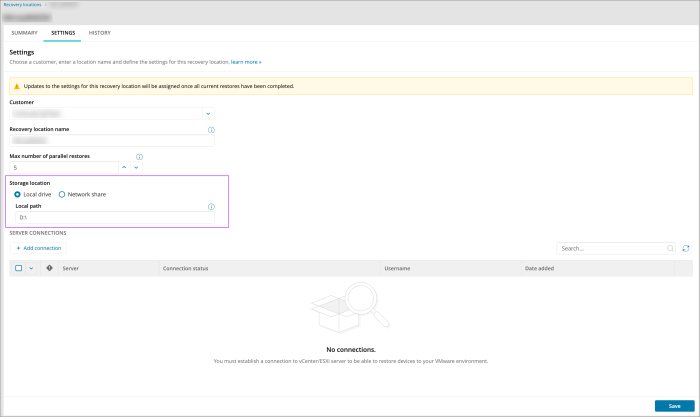The image displays an interface with a gray outline and a variety of elements. At the top, there's a gray box featuring blue text and several redacted sections. The background is white, with several items underlined in blue, including "Summary" and "Settings," which leads into items labeled "History" and another instance of "Settings" followed by descriptive text. 

A pink box with a yellow arrow appears, containing small print explaining updates to settings for recovery locations. Below this, there is a section labeled "Customer" with a search bar that is blanked out, followed by several fields such as "Recovery Location Name," "Max Number of Restores," and "Parallel Restores," all of which have blanked-out entries and accompanying search icons or up and down arrows.

Additionally, there is a purple-outlined box labeled "Storage Location," containing blue and white circular icons for "Local" and "Network Share" paths, accompanied by search functionality. This section also includes "Service Connections" and a button labeled "All Connections." 

Further down, there's a long gray box with a small blue box and blue downward arrow in the top corner, detailing sections for "Server and Connections," "Username," and an unspecified addition. In the background, a smaller box features a magnifying glass icon and the text "No connections," ending with a line and a prominent blue "Save" button.